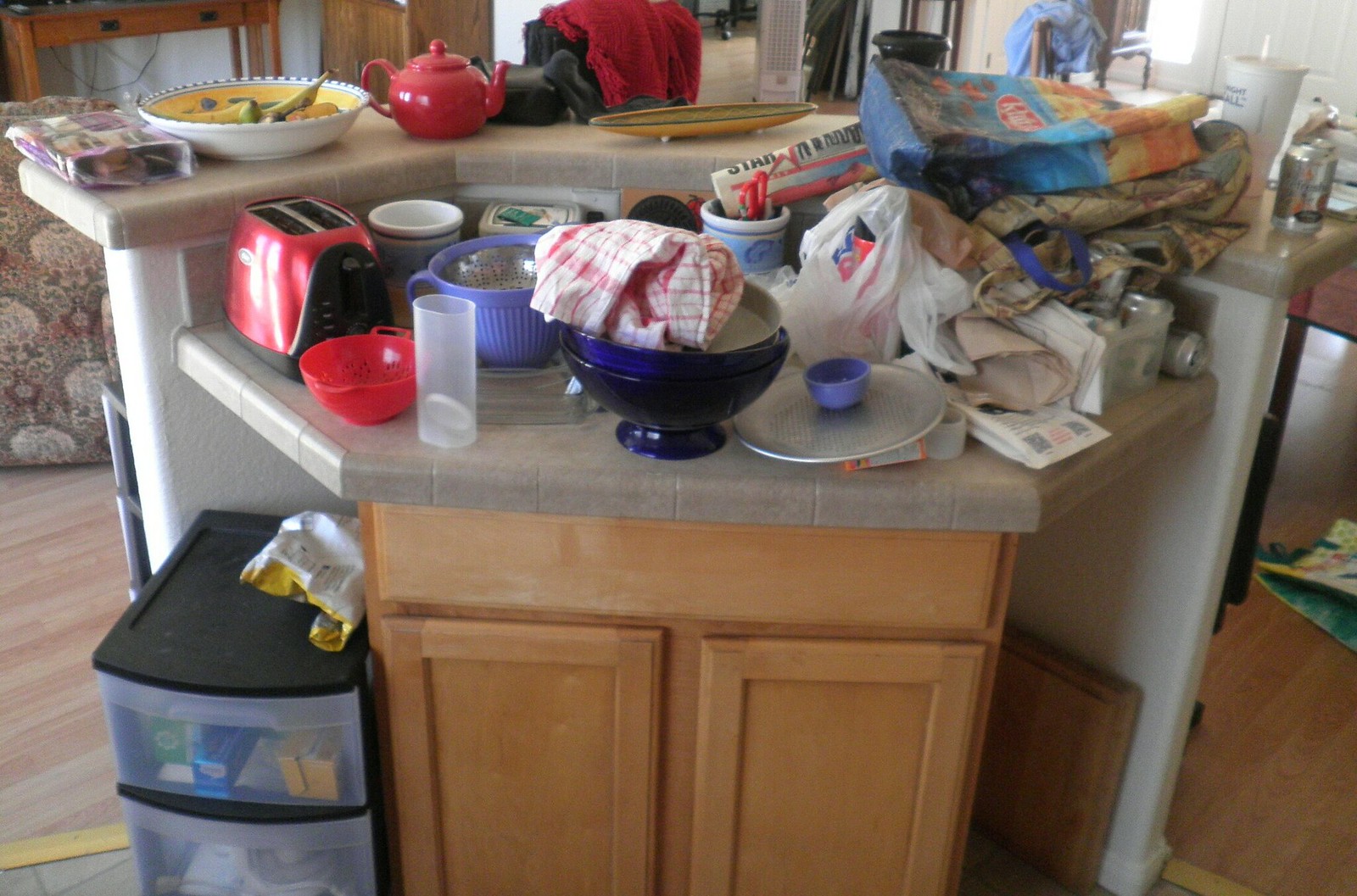A detailed description of the image reveals a cluttered kitchen scene. Along the back counter, a glass bowl filled with fruit is prominently displayed next to a package of cookies wrapped in plastic. A vibrant red teapot stands out among other items, which include what appears to be a piece of luggage draped with a sweater. Also on the counter is a lid, a shopping bag with text that suggests it might be a beach bag, a cup from a fast-food restaurant with a straw, and a can of soda or another beverage.

The kitchen counter itself seems to be part of an island setup. The front section of this island is equally cluttered, showcasing a red toaster, a red colander, a plastic container, a blue colander that nests a metal colander inside, a dish towel, a plastic shopping bag, a blue bowl with a lid nearby. Below the counter, two brown cupboards provide storage, while to their left, two plastic bins contain various items, including what looks like Reynolds wrap and cellophane. The overall scene paints a vivid picture of a busy, lived-in kitchen space bustling with various domestic items.